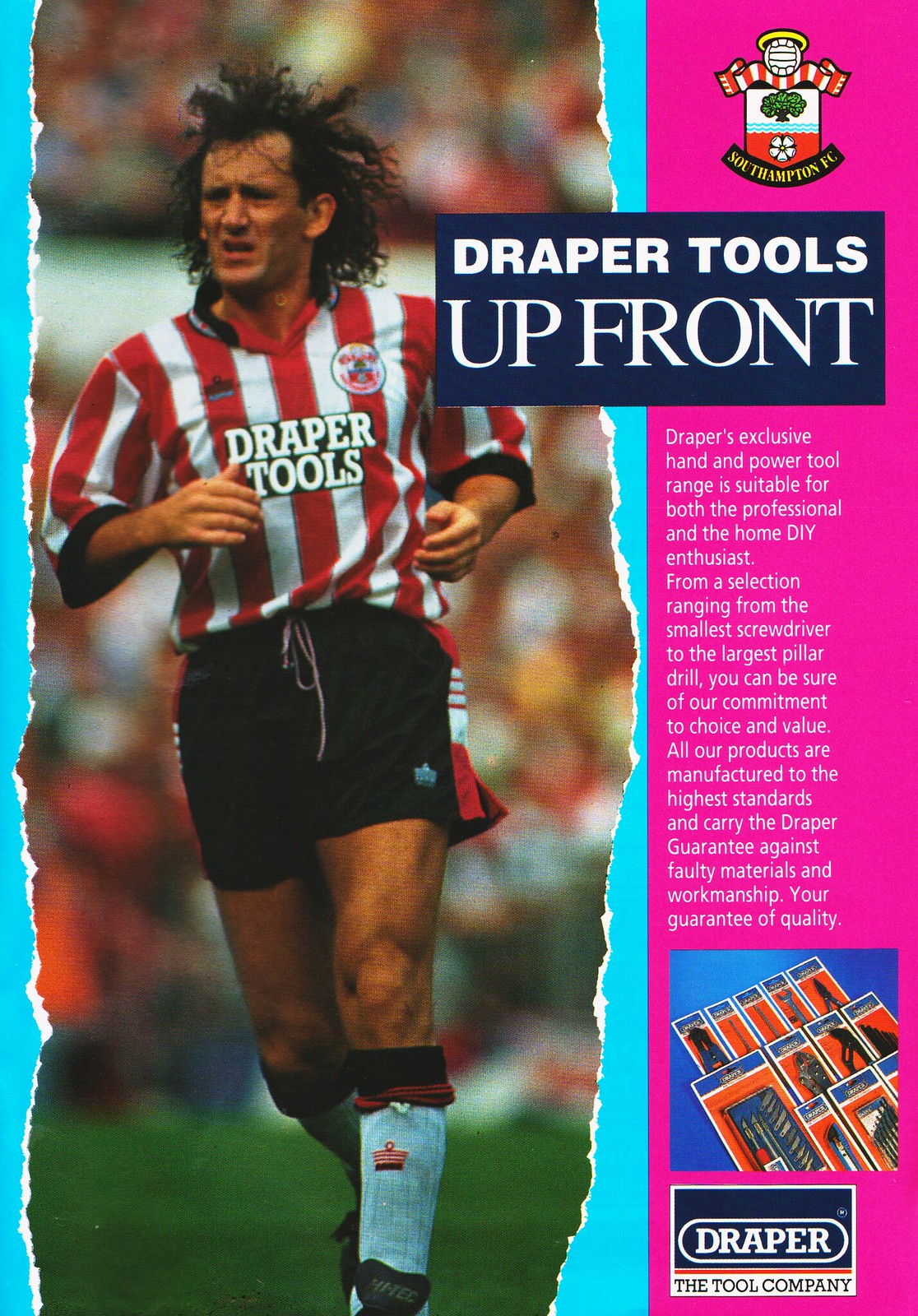The image is an advertisement featuring a soccer player believed to be from England. The player, a white male with long, curly dark hair, is depicted running on a field. He is dressed in a red and white striped shirt with "Draper Tools" printed in white on the front, accompanied by black shorts with red and white stripes down the side, and black and white knee socks. The player is positioned on the left-hand side of the image, which dominates the ad. On the right-hand side, there is a crest labeled "Southampton FC" in the upper right corner. Below this is a blue square with the text "Draper Tools up front" in white letters, followed by smaller white text detailing Draper's exclusive hand and power tool range. Further down, there's a square image with a blue background showing stacked trading cards or tools in plastic. At the bottom, there is a white square featuring a blue square inside, where it says "Draper" and below that "The Tool Company." The entire composition promotes Draper Tools through the sponsorship of the athlete’s soccer team.